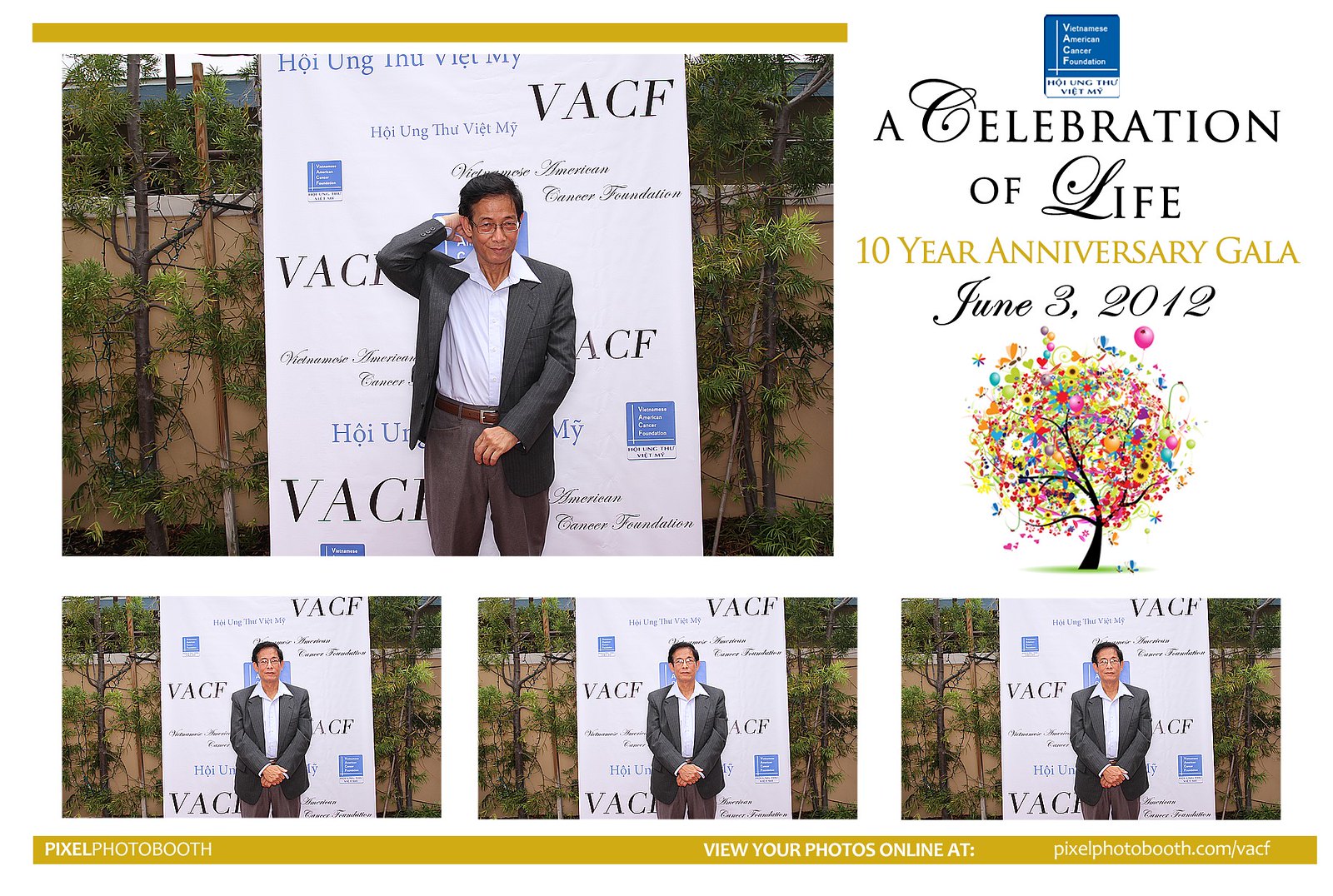The image is a collage featuring a total of four photographs. At the top left is a large photograph of a middle-aged Asian man with tanned brown skin and black hair, wearing glasses. He is dressed in a dark gray blazer, a white 70s-style button-up shirt with the collar out, dark brown pants, and a brown belt. In this photo, he is posing with one hand up to his ear and the other by his waist. Behind him is a vertical white banner covered in various logos and foreign text, likely Chinese or Korean, along with the acronym VACF displayed prominently multiple times in black font. The backdrop includes thin trees with sparse green leaves and a light brown wall extending across the image. 

Below this large photograph, the same man is seen in three smaller, repeated photographs at the bottom of the collage, identical in outfit and background but posing differently with both hands to his waist area. 

In the top right corner of the image, text reads "A Celebration of Life" in black and gold, followed by "10-Year Anniversary Gala" and the date "June 3, 2012." Adjacent to this text is a blue square logo with "Vietnam American Cancer Foundation" written in white font. There is also a colorful cartoon illustration of a tree with leaves in various colors, including yellow, red, pink, blue, and green.

At the very bottom of the collage, a yellow stripe contains the text "Pixel Photo Booth," followed by "View your photos online at pixelphotobooth.com/vacf" in white font.